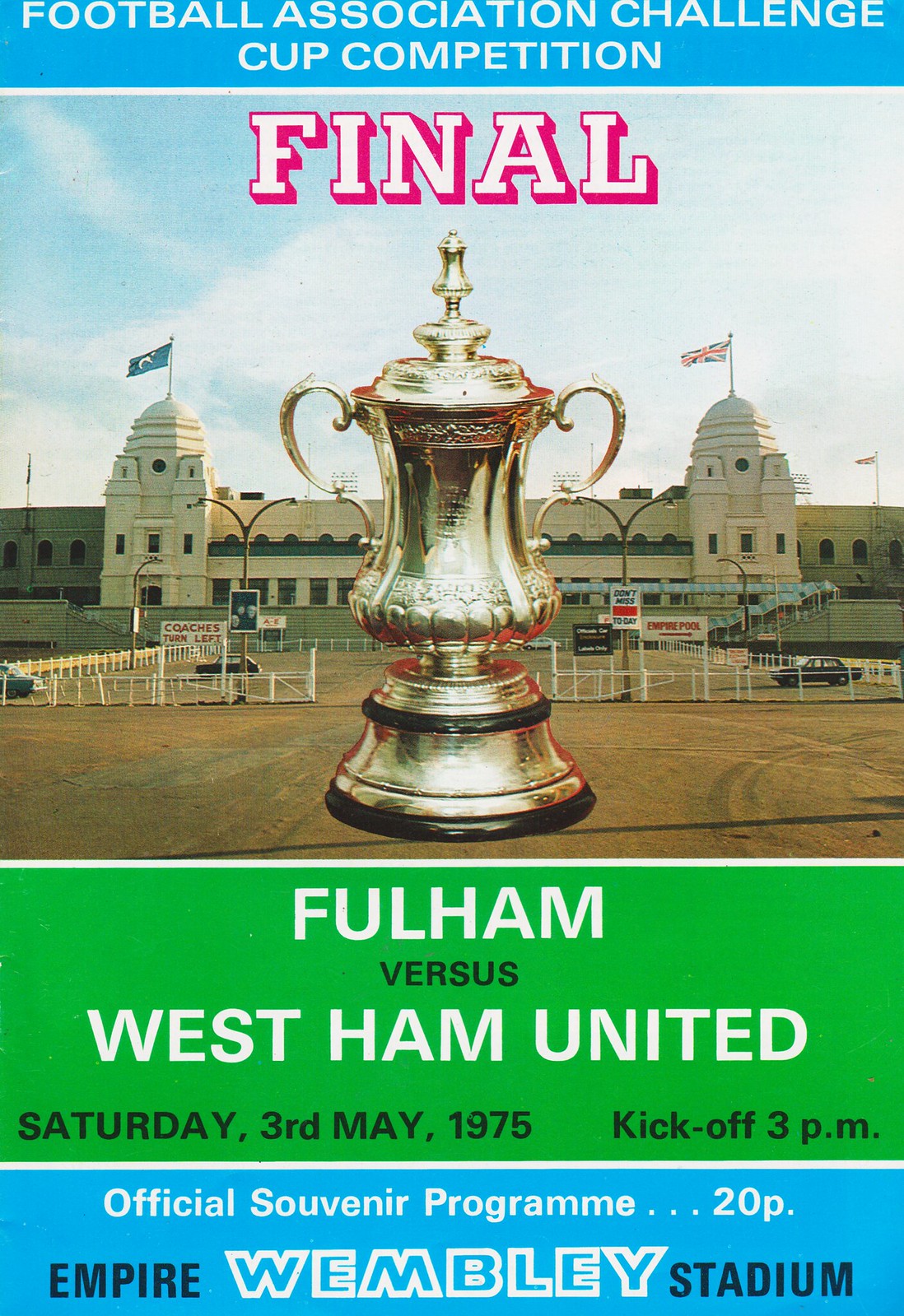This image is a detailed advertisement and program cover for the 1975 Football Association Challenge Cup Final featuring Fulham versus West Ham United. The layout is horizontally aligned into four panels. At the top, a blue banner displays "FOOTBALL ASSOCIATION CHALLENGE" in uppercase white letters, followed by "CUP COMPETITION" centered beneath it, and a thin white line underneath.

The central panel contains a photographic backdrop of the iconic Wembley Stadium, characterized by two dome-like structures on either side with flags, possibly from the Middle East, fluttering atop them. These buildings have distinct architecture featuring towers, multiple windows, and columned lower sections with wavy designs. The foreground displays a dry, earthy ground with patches of grass near the buildings, white fencing, and a sign with red writing to the right. Prominently positioned in the middle is a large, ornate cup with an elaborate design, curly handles, and multiple circular layers atop it. "FINAL" is set in bold white letters over a pink block, centered across the photograph.

Beneath the photograph, a green panel includes essential match details: "FULHAM" in large uppercase white letters followed by "vs" in smaller black uppercase letters and "WEST HAM UNITED" again in large uppercase white. Extending further along the bottom in black text are "SATURDAY 3RD MAY, 1975," "KICKOFF 3 PM," and two thin white lines marking the panel's boundaries.

The final blue panel at the bottom reads "OFFICIAL SOUVENIR PROGRAMME 20P" in centered white text, followed by "EMPIRE-WEMBLEY STADIUM," emphasizing the historic British location.

This program cover effectively combines crucial event information with a rich visual representation of the stadium, reinforcing the significance of the 1975 cup final between Fulham and West Ham United.